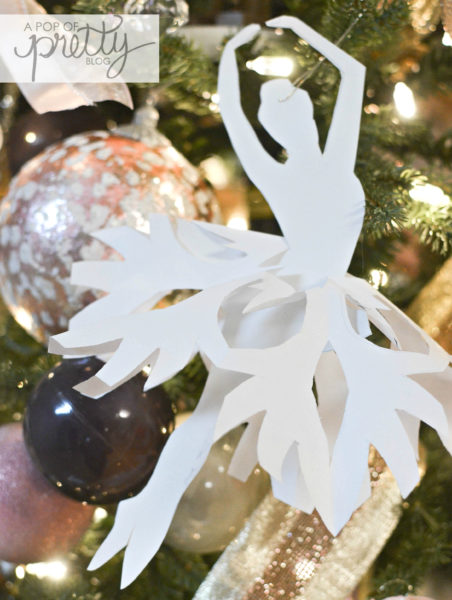The image features a detailed close-up of a decorated Christmas tree, showcasing a variety of colorful ornaments and festive lights. The centerpiece is an intricate white paper cutout of a ballerina, her dress designed to resemble a snowflake with a 3D effect. She is captured in a classic ballet pose, with arms gracefully arched above her head and toes pointed downward. The ballerina ornament is attached to the tree with a silver clasp. Around her, the lush green pine needles of the tree are adorned with several ornaments: a white and silver ornament speckled with white, a glassy black bauble, a glittery purple globe, and a clear shiny decoration. The tree is also illuminated with small white lights, enhancing its festive appeal. In the upper left corner, a white rectangle displays the text "a pop of pretty blog," with "pretty" written in cursive.